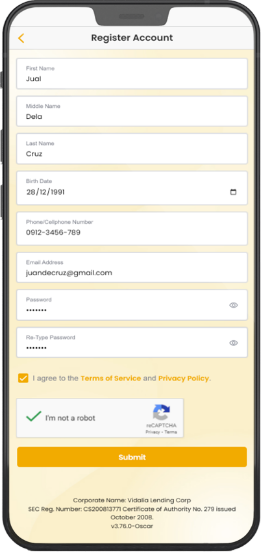This image depicts a mobile phone displaying a registration form within a black-outlined, multi-colored case featuring a light tan, gray, and white color scheme. At the top of the screen, a gray banner stretches across with "Register Account" boldly written in black. On the left side of the banner, there is a left-pointing orange triangle symbol.

Below the banner, the form consists of several rectangular white fields, each labeled in black. The first field is labeled "First Name" with the entered name "J-U-A-L." The second line is labeled "Middle Name," showing "D-E-L-A," and the third line is labeled "Last Name" containing "Cruz" in black text. Next, the "Birth Date" field is filled with "28-12-1991," accompanied by a calendar icon on the far right.

Further down, the form asks for a phone number and an email address, each presented in bold black, though specific details are generalized here. The "Password" field contains seven asterisks, with a grayed-out eyeball icon situated on the right, indicating a hidden password option. The subsequent "Retype Password" field mirrors this format, also displaying seven asterisks with an eyeball icon on the right.

Beneath these fields, against a tan background, an orange-checked square indicates agreement to the "terms and service and privacy policy." Following this, a white CAPTCHA section with a capital "C" that is blue on top and a green-checkmarked "I am not a robot" box appears prominently. At the bottom of the form, an orange bar with yellow text reads "Submit."

Finally, towards the bottom of the image, the corporate name "Medallia Lending Corp." appears, followed by an SEC registration number, adding a final touch of formality to the screenshot.